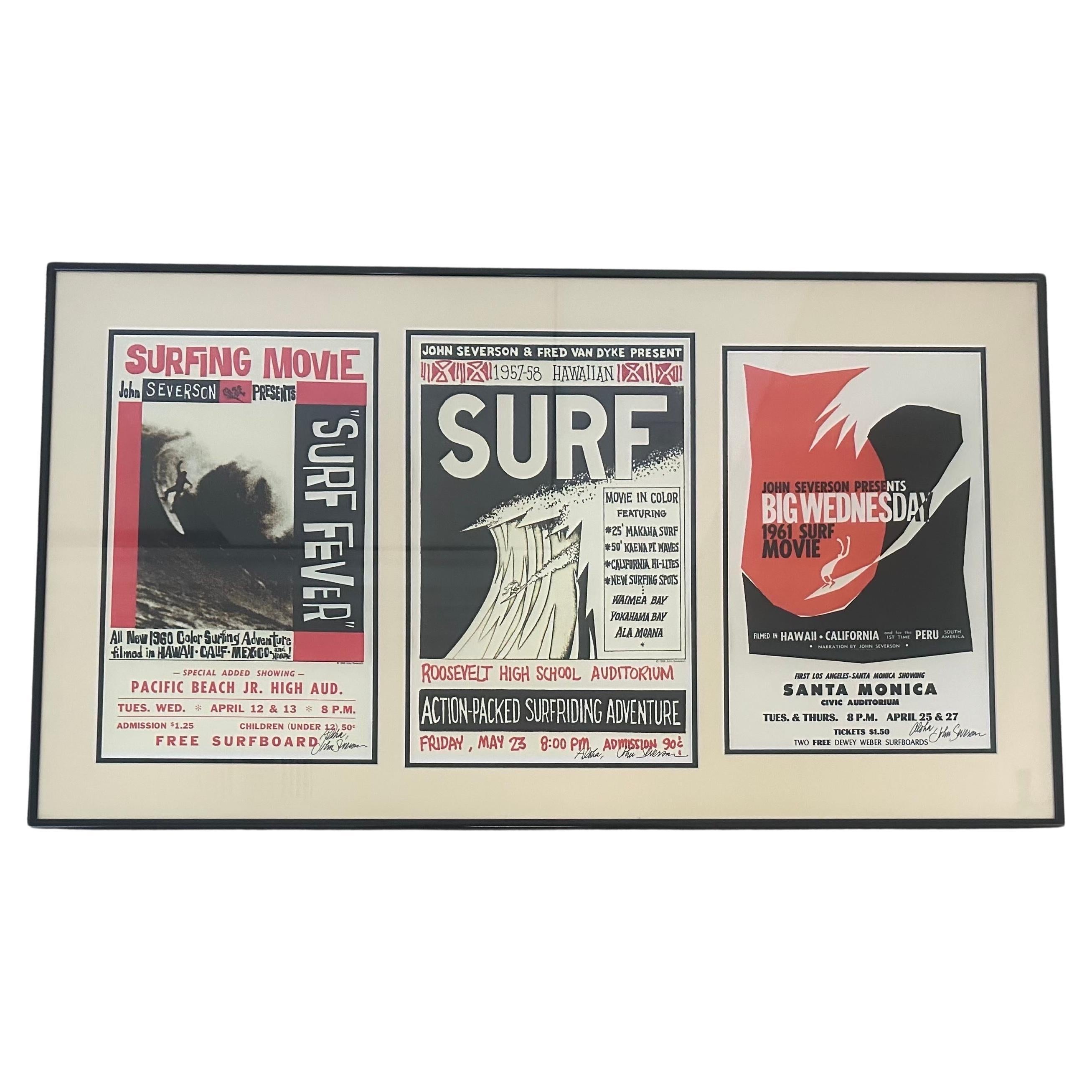This is a photograph of a framed set of three surf movie posters, meticulously arranged in a single black frame with a white mat. Each poster, marked by various shades of red, white, and black, prominently features signatures in the bottom right-hand corner. 

The first poster, titled "Surf Fever," advertises a 1960 color surfing adventure presented by John Severson. This film was shot in Hawaii, California, and Mexico, with a special showing at the Pacific Beach Junior High Auditorium on April 12th and 13th at 8 p.m. Admission is $1.25 for adults and 50 cents for children under 12, with a free surfboard giveaway included.

The central poster promotes the 1957-58 Hawaiian Surf, a movie presented by John Severson and Fred Van Dyke. It highlights captivating scenes of 12-foot Makaha surf, 50-foot Kahuna waves, and new surfing spots at Waimea Bay, Yokohama Bay, and Ala Moana. This action-packed film is set to be shown at Roosevelt High School Auditorium on Friday, May 23rd at 8 p.m., with an admission fee of 90 cents.

The final poster, "Big Wednesday," is presented by John Severson and features a 1961 surf movie filmed in Hawaii, California, and Peru. This poster, with its striking design of a white surf against a red background, announces showings at the Santa Monica Civic Auditorium on April 25th and 27th at 8 p.m. Tickets are priced at $1.50, and the screening includes a chance to win two free Dewey Weber surfboards.